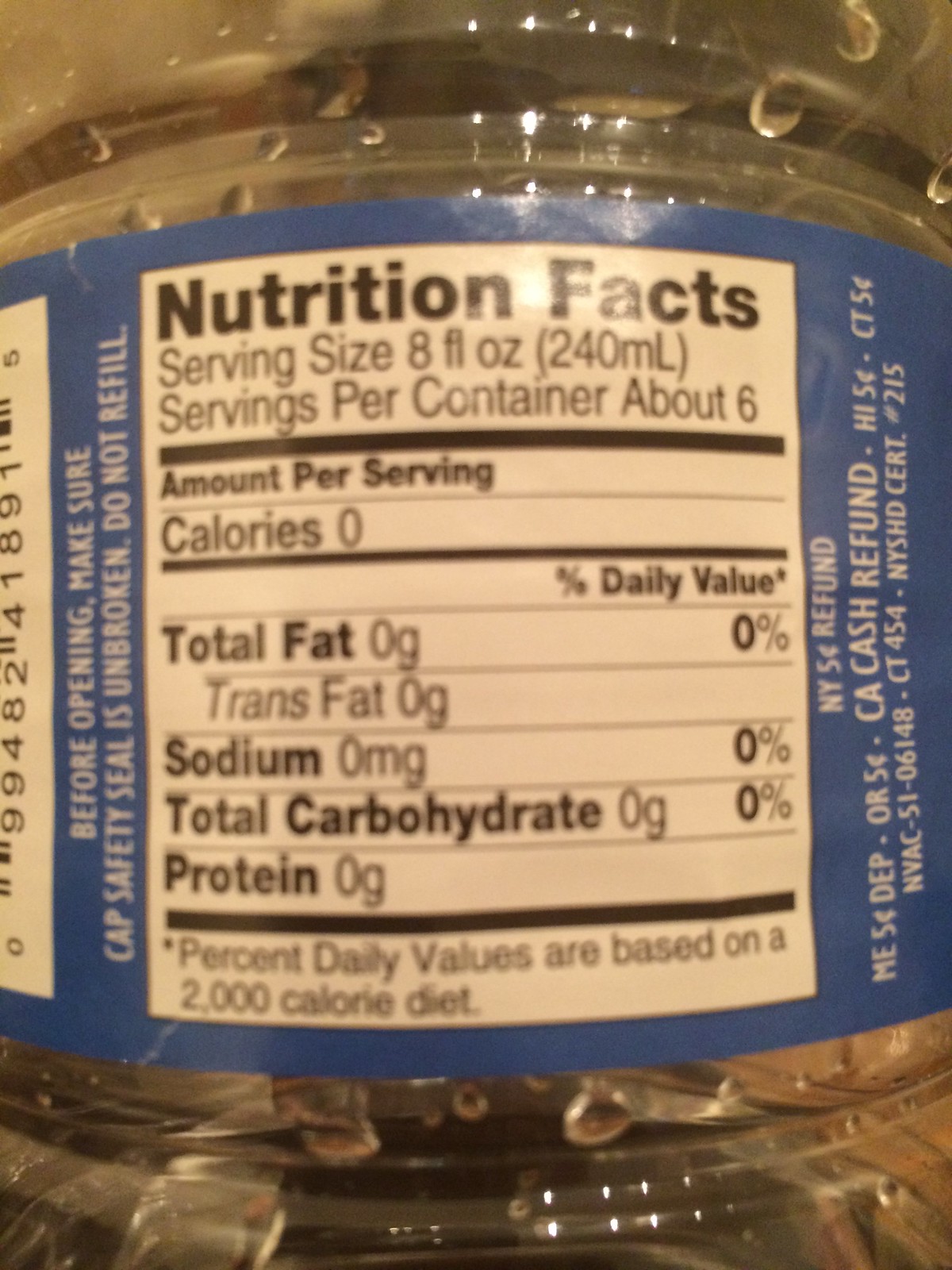The image shows a close-up view of the back of a clear water bottle with visible water droplets inside. The bottle is labeled with a blue nutrition facts panel featuring white and black text. The nutrition facts read: "Serving Size: 8 fluid ounces (240 mL)," "Servings Per Container: About 6," "Calories: 0," "Total Fat: 0 grams (0% DV)," "Trans Fat: 0 grams," "Sodium: 0 milligrams (0% DV)," "Total Carbohydrates: 0 grams (0% DV)," and "Protein: 0 grams." A note mentions that the percent daily values are based on a 2,000 calorie diet. Additionally, there is small white text on the blue label advising, "Before opening, make sure cap safety seal is unbroken. Do not refill." On the right side of the label, it lists various state-specific refund values: "New York - 5 cent refund," "Maine - 5 cent," "DEP-OR - 5 cent," "CA Cash Refund," "HI - 5 cent," and Connecticut 5 cent. Some edges of a barcode and various certification codes are also partially visible on the left side of the label.